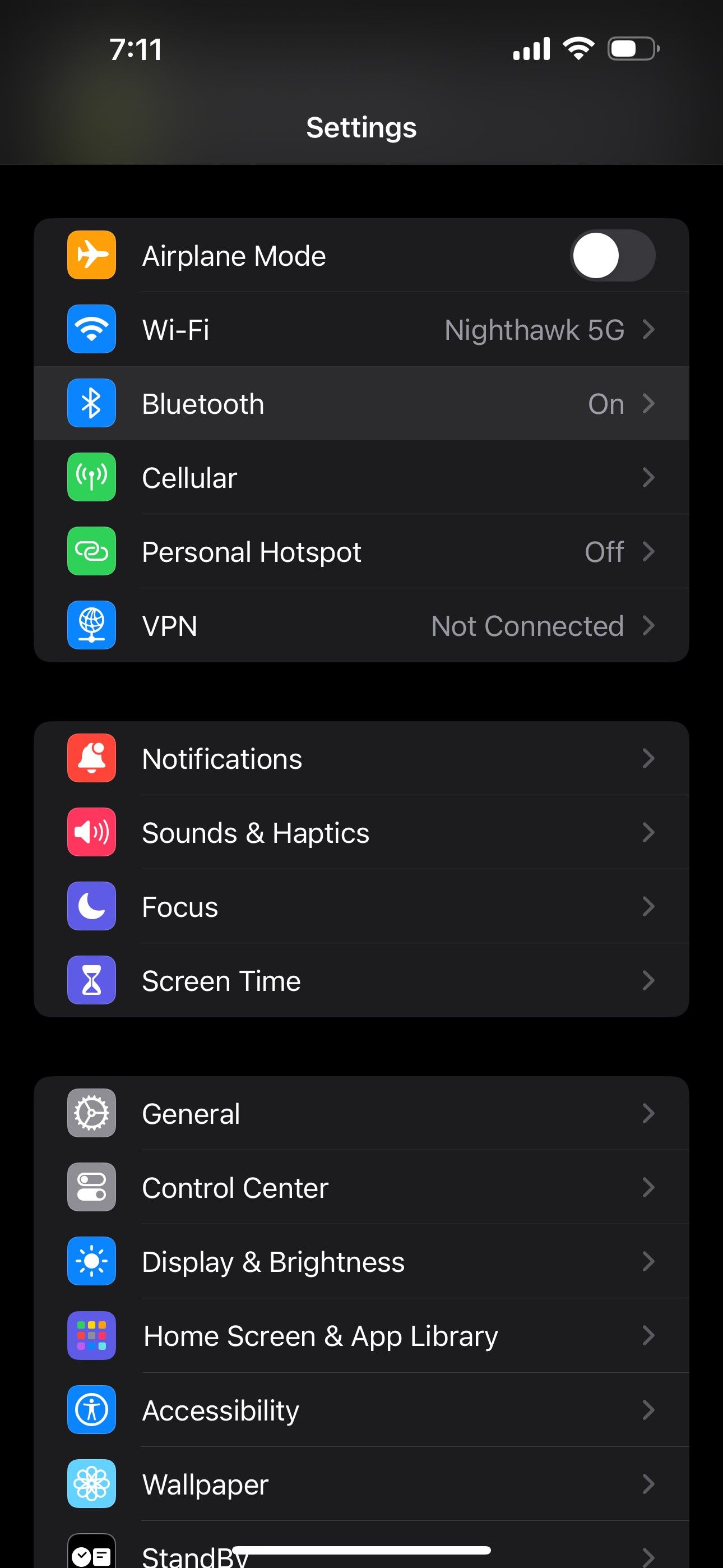The screenshot depicts the Settings page of an iPhone in Dark Mode. The interface is shown against a dimly-lit background, providing a clear contrast to the white text. 

In the top left corner, the time is displayed as "7:11." In the top-right corner, various indicators show the device's status: the battery is at approximately 75% charge, Wi-Fi is fully connected, and the signal strength is at its maximum.

Centered near the top, the word "Settings" is written in white, slightly below the top header. The settings menu is organized into different sections, each with corresponding icons to the left and a gray caret on the right, except for "Airplane Mode," which features a toggle switch that is currently turned off.

The first section lists:
1. **Airplane Mode** (with a toggle switch, currently off)
2. **Wi-Fi**
3. **Bluetooth**
4. **Cellular**
5. **Personal Hotspot**
6. **VPN**

The second section includes:
1. **Notifications**
2. **Sounds & Haptics**
3. **Focus**
4. **Screen Time**

The third section consists of:
1. **General**
2. **Control Center**
3. **Display & Brightness**
4. **Home Screen & App Library**
5. **Accessibility**
6. **Wallpaper**
7. **Standby**

Each section is distinctly separated, ensuring easy navigation through the various settings options.